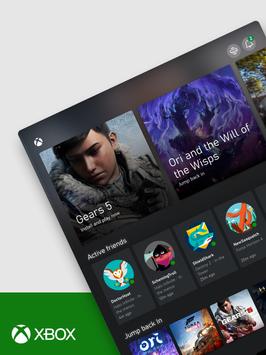The image portrays a vertically oriented display that is approximately 30 to 50 percent taller than it is wide. The overall background features a medium gray tone, giving it a neutral and unobtrusive appearance. At the bottom, occupying about 15 to 20 percent of the total image height, there is a striking grass-green banner. This banner sports the recognizable Xbox logo on the lower left corner, along with the word "Xbox" prominently displayed in white text. 

Overlaying this backdrop is a depiction of a mobile interface positioned diagonally, starting from the lower right-hand corner and slanting towards the upper left, aligned at roughly 10:30 to 11 o'clock. This mobile page is truncated at the right and bottom edges, suggesting a focus upwards into the image. The mobile interface itself has a dark gray background and is populated with clickable article previews, likely from Xbox’s recent showcase. Featured at the top of this page is content related to "Gears 5" in the upper left corner, followed by "Ori" below it. In addition, there is an active friends area that indicates a user is logged in, enhancing the interactive and personal touch of the presentation.